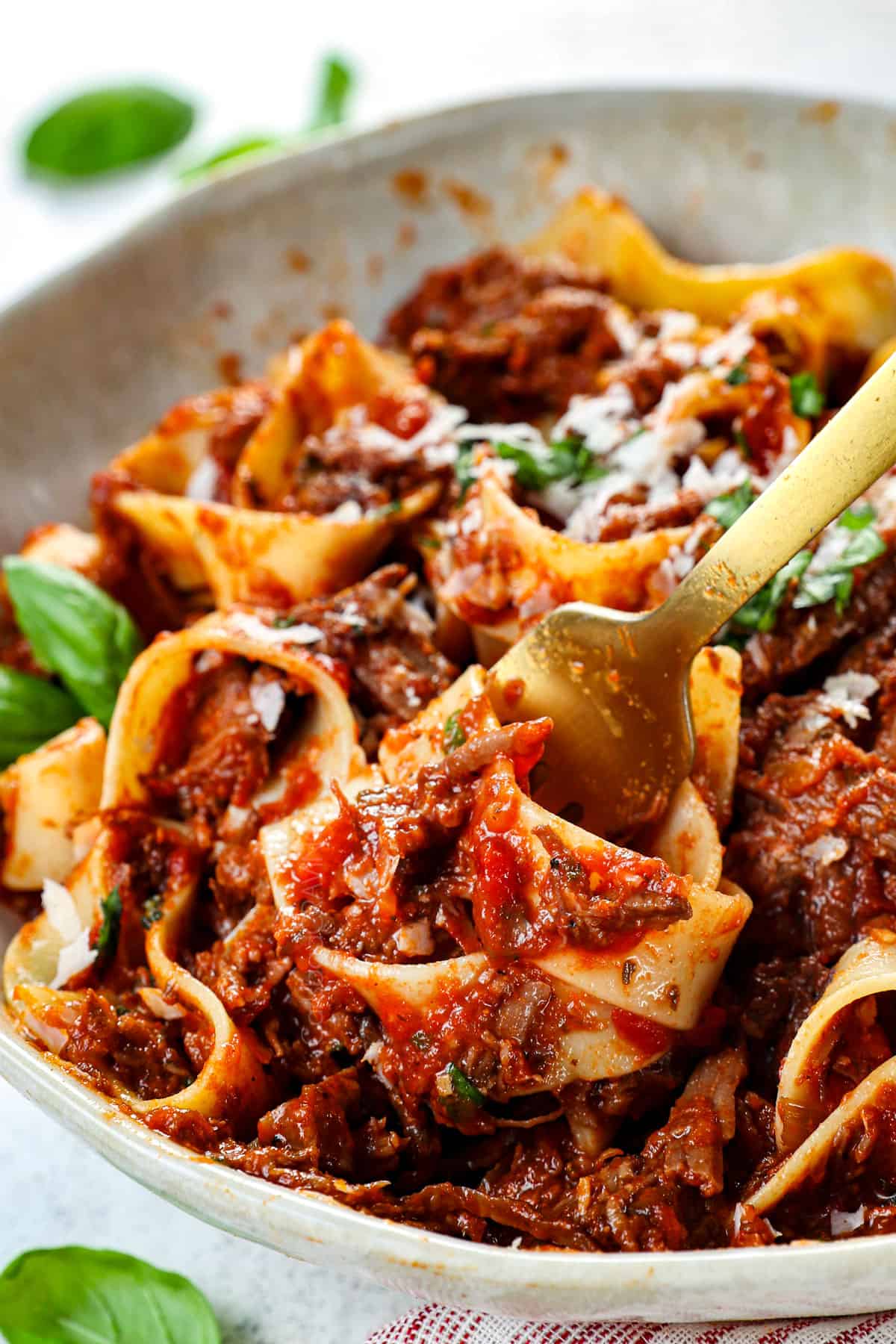In this high-quality image, we see a white bowl or plate filled with a visually appetizing pasta dish. The pasta, featuring flat noodles, is generously coated with a vibrant red tomato-based sauce. Interspersed among the noodles are chunks that appear to be ground beef, adding hearty texture to the dish. A golden or silver fork is elegantly placed within the pasta, capturing a bite. 

Topping the pasta, there is a sprinkling of white cheese, likely Parmesan, along with fresh green basil and parsley leaves. The surface under the bowl appears to be a marble table, adding a touch of sophistication, with a glimpse of red and white napkins at the bottom edge. Additionally, the image is adorned with fresh basil and parsley leaves scattered around the upper and lower left corners, complementing the dish's garnish. The detailed textures and vibrant colors make this pasta dish look especially delectable.